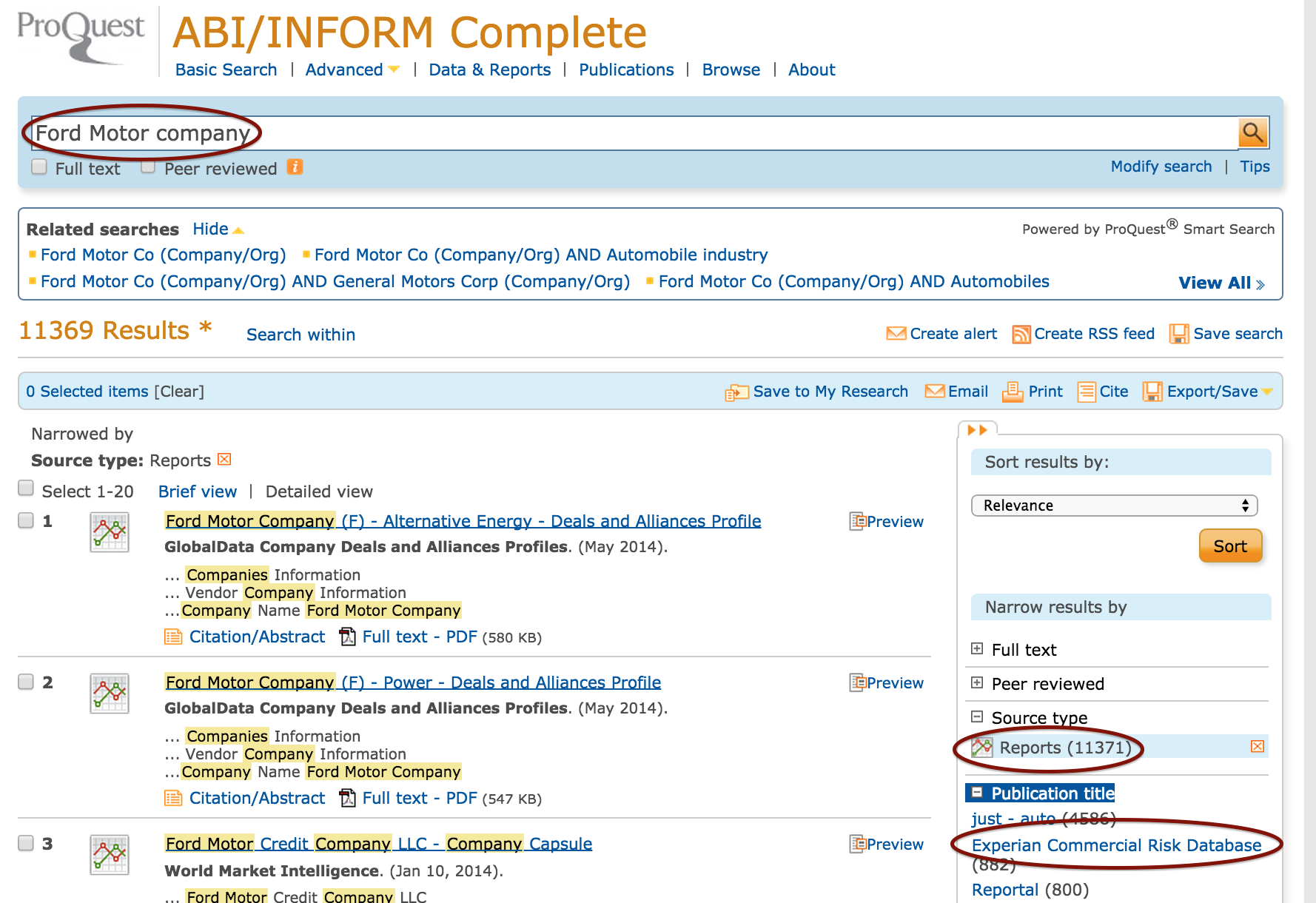This detailed screenshot from the ProQuest ABI/INFORM Complete database interface shows a search for "Ford Motor Company". At the top of the screen, navigation options include Basic Search, Advanced Data and Reports, Publications, Browse, and About. The search term "Ford Motor Company" is entered in the search bar and circled for emphasis.

Various search options and filters are visible, such as Full Text, Peer-Reviewed, Modify Search, and Related Searches. The search results are generated through ProQuest Smart Search, yielding a total of 11,371 results, with search options to view all, search within results, create an alert, and create an RSS feed. Features to save the search, email, print, cite, and export results are also available.

The results are presented in both brief and detailed view formats. The top three results include:

1. "Ford Motor Company: Alternative Energy Deals and Alliances Profile" by GlobalData Company, from May 2014, available in full text and PDF (580 KB).
2. "Ford Motor Company (F): Power Deals and Alliances Profile" by GlobalData Company, from May 2014, available in full text and PDF (547 KB).
3. "Ford Motor Credit Company, LLC: Company Capsule" by World Market Intelligence, from January 10, 2014.

On the right side of the screen, a vertical menu offers sorting options by relevance, and narrowing results by Full Text, Peer-Reviewed, and Source Type. The selected Source Type is "Reports" with a count of 11,371 results, highlighted and circled. The Publication Titles included are "Just Auto" with 4,586 entries, "Experian Commercial Risk Database" with 882 entries (circled), and "Reportal" with 800 entries.